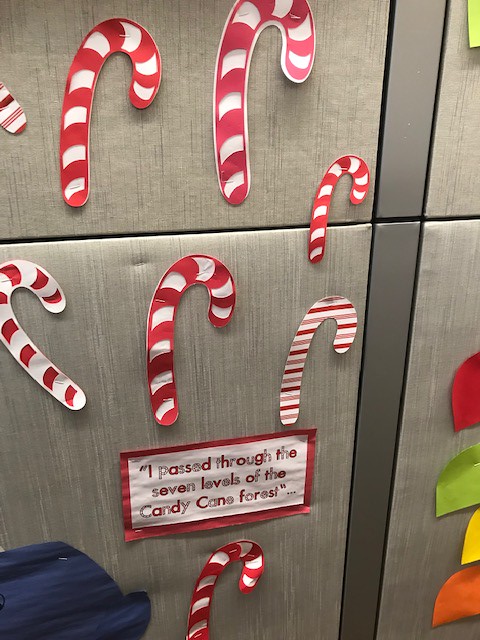The image depicts an office wall adorned with an array of hand-cut paper candy canes, illustrating a whimsical scene. The majority of the candy canes feature traditional red and white stripes, while a few are predominantly white with red accents. These decorations are stapled to a spongy, vinyl-like material, creating a soft-textured backdrop. At the bottom of the display, a cut-out paper sign reads, "I passed through the seven levels of the candy cane forest," enclosed in parentheses. Surrounding these candy canes are additional colorful paper cutouts resembling leaves in hues of red, green, yellow, and orange. The bottom right corner of the image hints at a blue object, possibly a trash can, partially visible and adding a contrasting element to the festive decor.